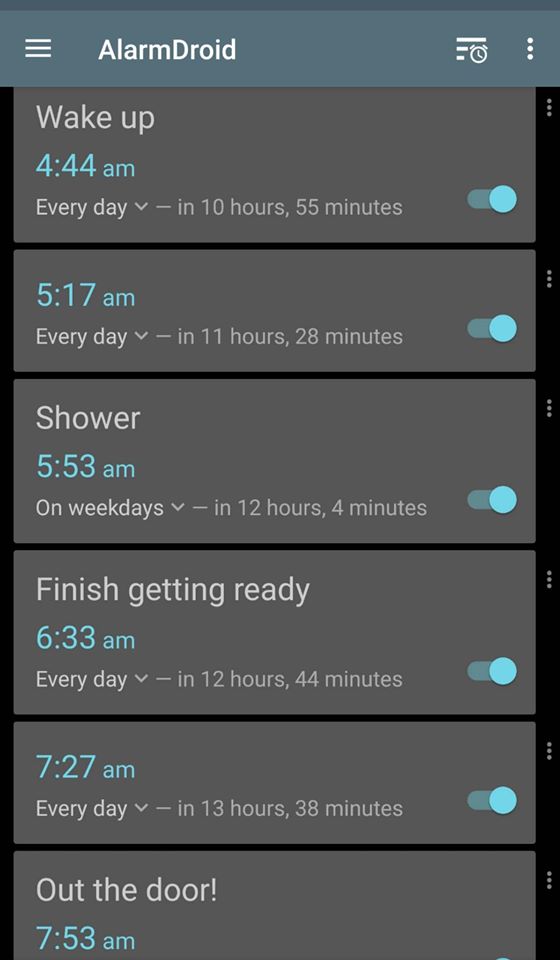The screenshot appears to capture the interface of an alarm management app, possibly named "Alarm Droid." The layout is predominantly in portrait orientation. In the upper left corner, there are three white horizontal bars representing a menu icon. To the far right of this icon, another set of three horizontal lines forms a vector graphic resembling an alarm clock. Further to the right, three vertically stacked dots denote additional options.

The main section of the screenshot is divided into six distinct rows, each row representing a different scheduled event or alarm. Each row contains various details and a radio button to its right, indicating whether the alarm is active:

1. **Wake Up:**
   - Time: 4:44 a.m. every day
   - Countdown: 10 hours, 55 minutes
   - Status: Radio box on the right
   - Additional: Ellipses to the upper right outside the rectangle

2. **Alarm 2:**
   - Time: 5:17 a.m. every day
   - Countdown: 11 hours, 20 minutes
   - Status: Radio button on the right

3. **Shower:**
   - Time: 5:53 a.m. on weekdays
   - Countdown: 12 hours, 4 minutes
   - Status: Radio button on the right

4. **Finish Getting Ready:**
   - Time: 6:33 a.m. every day
   - Countdown: 12 hours, 44 minutes
   - Status: Radio button on the right

5. **No Title:**
   - Time: 7:27 a.m. every day
   - Countdown: 13 hours, 38 minutes
   - Status: No title associated with this time

6. **Out the Door:**
   - Time: 7:53 a.m.
   - Details of the bottom rows are truncated in the screenshot

Overall, the interface seems organized with a clean look, providing clear visibility of each alarm's time, frequency, countdown, and activation status. The truncation at the bottom suggests there might be additional alarms or options that are not visible in the current view.